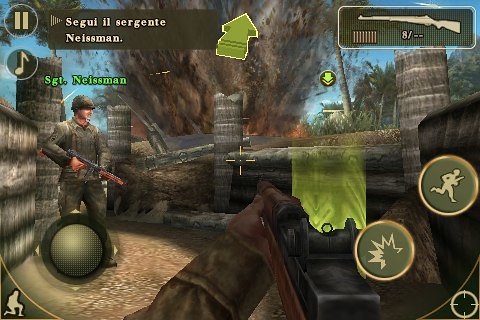This image is a detailed screenshot from a first-person shooting video game, exhibiting various gameplay controls and HUD elements. The player's perspective shows them holding a shotgun, partially obscured by a brownish-green shirt and brown glove or potentially brown skin. The setting features a trench-like area with trees visible in the background.

The bottom left corner displays a kneeling silhouette, likely indicating the player’s character position. Adjacent to it on the right is an ambiguous circular graphic. The bottom right corner comprises a target icon and a green circular icon with a gold rim and a pale brown center, depicting an explosion. Above it, a similar circular icon shows a running man with a gun, presumably for sprint controls.

Prominent details include another player, Sergeant Nisman, positioned to the left, identifiable by the bright green text "Sgt. Nisman" above his head. The top left corner instructs "Segui il Sargente Nisman," which translates to "Follow Sergeant Nisman," and features circular buttons for pause and music controls. The top right corner provides ammunition information for the shotgun, displayed against a green background with vertical lines, indicating "8/--".

Overall, the predominant color theme involves army green, gold, and brown hues, complementing the camouflage outfits and rugged environment shown in the game.